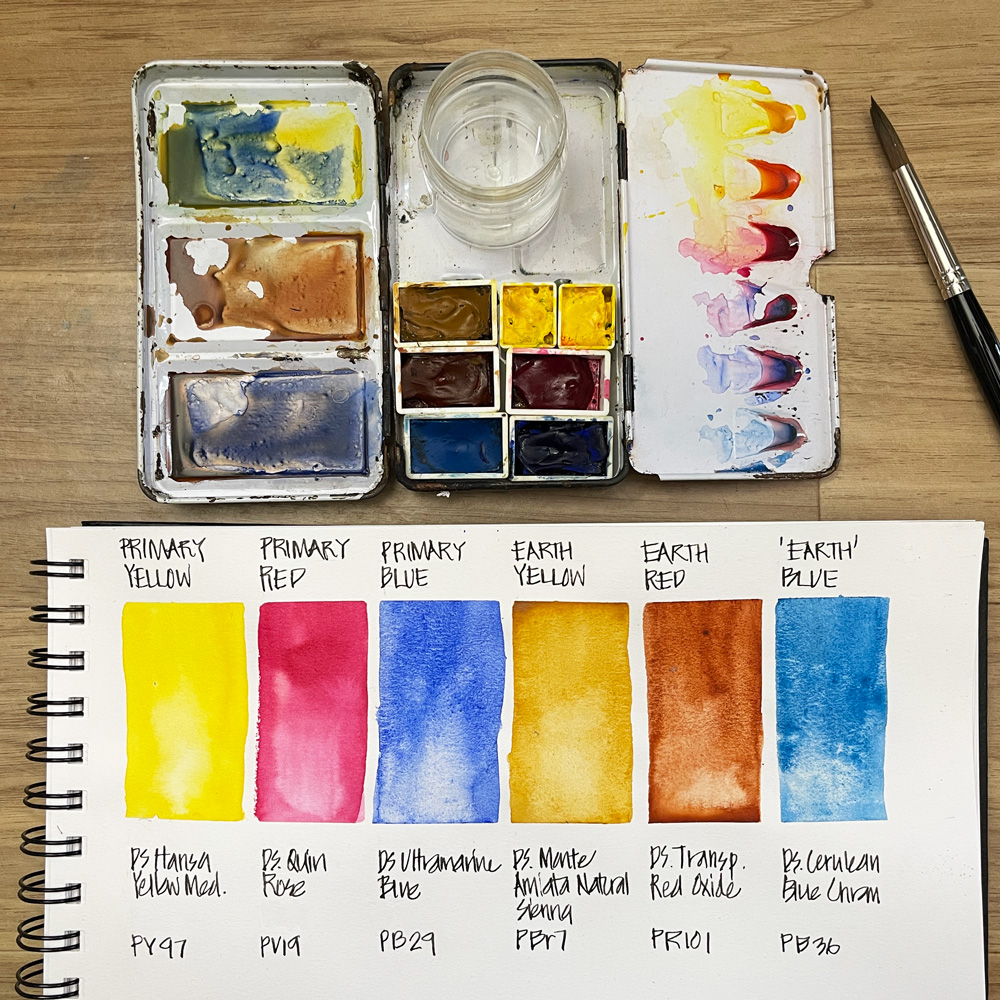The overhead photograph captures a detailed workspace setting on a brown wooden table. The top half showcases a white, foldable watercolor palette with three sections. The middle section holds a clear glass jar filled with water, while the left section contains three slots for solid watercolor paints. The right section features a watercolor brush and additional paint containers, with various mixed hues of yellow, brown, blue, and pinks visible in the palette.

The bottom half of the image displays a white spiral-bound sketchbook opened flat, revealing six vertical rectangular swatches of watercolors, meticulously labeled with their respective names and color codes. From left to right, the swatches are: 

1. **Primary Yellow** - DS Hansa Yellow Medium (PY 97), featuring a bright yellow block.
2. **Primary Red** - DS Quinacridone Rose (PV 19), showcasing a vivid red block.
3. **Primary Blue** - DS Ultramarine Blue (PB 29), presenting a deep blue block.
4. **Earth Yellow** - DS Monte Amiata Natural Sienna (PBR 7), a darker, earthy yellow block.
5. **Earth Red** - DS Transparent Red Oxide (PR 101), appearing more like a brownish-red block.
6. **Earth Blue** - DS Cerulean Blue Chrome (PB 36), a lighter blue compared to the primary blue.

Each swatch is clearly labeled with detailed color codes and technical descriptions, creating a comprehensive and organized display of watercolor options.